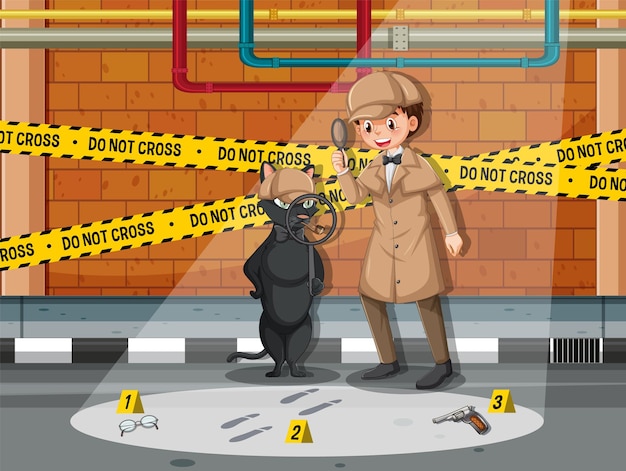In the image, a cartoon-style detective scene unfolds featuring two characters keen on solving a mystery. At the center stands a young boy dressed in a brown trench coat, brown pants, black shoes, and a brown detective hat. He holds a gray magnifying glass and wears a determined expression. Beside him is his assistant, a serious-looking cat dressed similarly in a brown hat, a gray bow tie, and a gray pipe in his mouth. The cat is also holding a magnifying glass.

They are investigating a crime scene marked by yellow "do not cross" tape that stretches in front of a brick wall adorned with colorful pipes. On the ground, three numbered placards identify critical clues: a pair of glasses labeled "1," two sets of footprints labeled "2," and a pistol labeled "3." The scene captures the essence of a classic detective investigation, complete with distinct characters, evident clues, and an air of suspense.